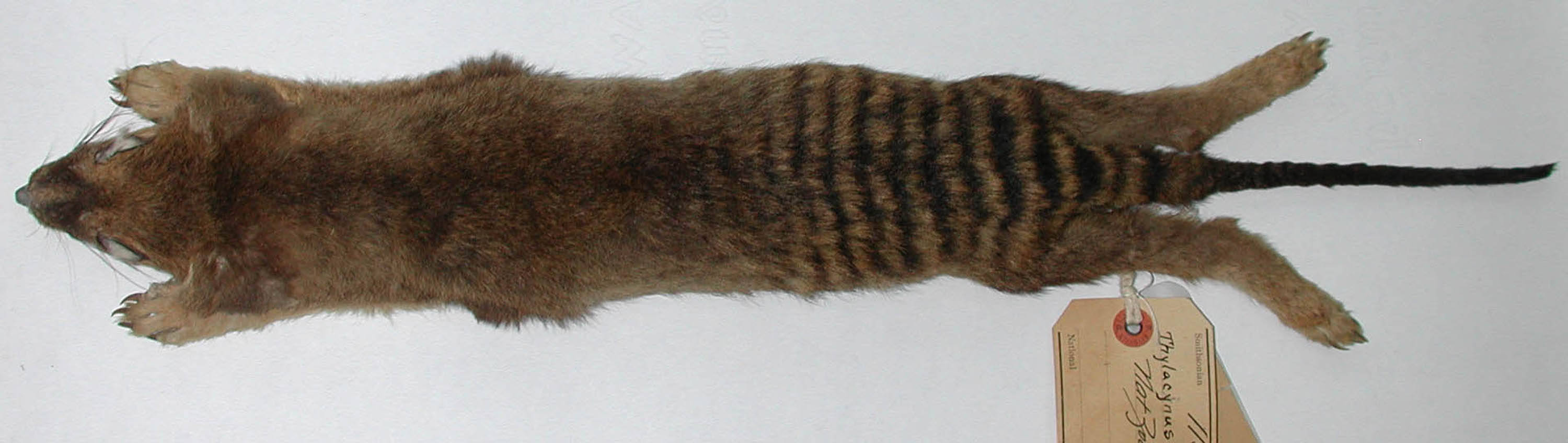This detailed, horizontally-oriented photograph captures the preserved skin of a small, unidentified animal, potentially a thylacine or similar creature. The animal is arranged flat on a white surface, with its front paws stretched out to the left and its back paws to the right. The fur is primarily brown, adorned with distinctive black stripes along the back half of its body. A long, black, and slender tail extends from its rear end. The animal's face is pointed and features whiskers, while its front paws display clear claws. Attached to one of its legs is a rectangular, old-looking paper tag with partially legible black printing and a red circle, spelling out "THYLACYNUS." The overall setting includes a gray background, emphasizing the animal’s prominently thin and elongated body.